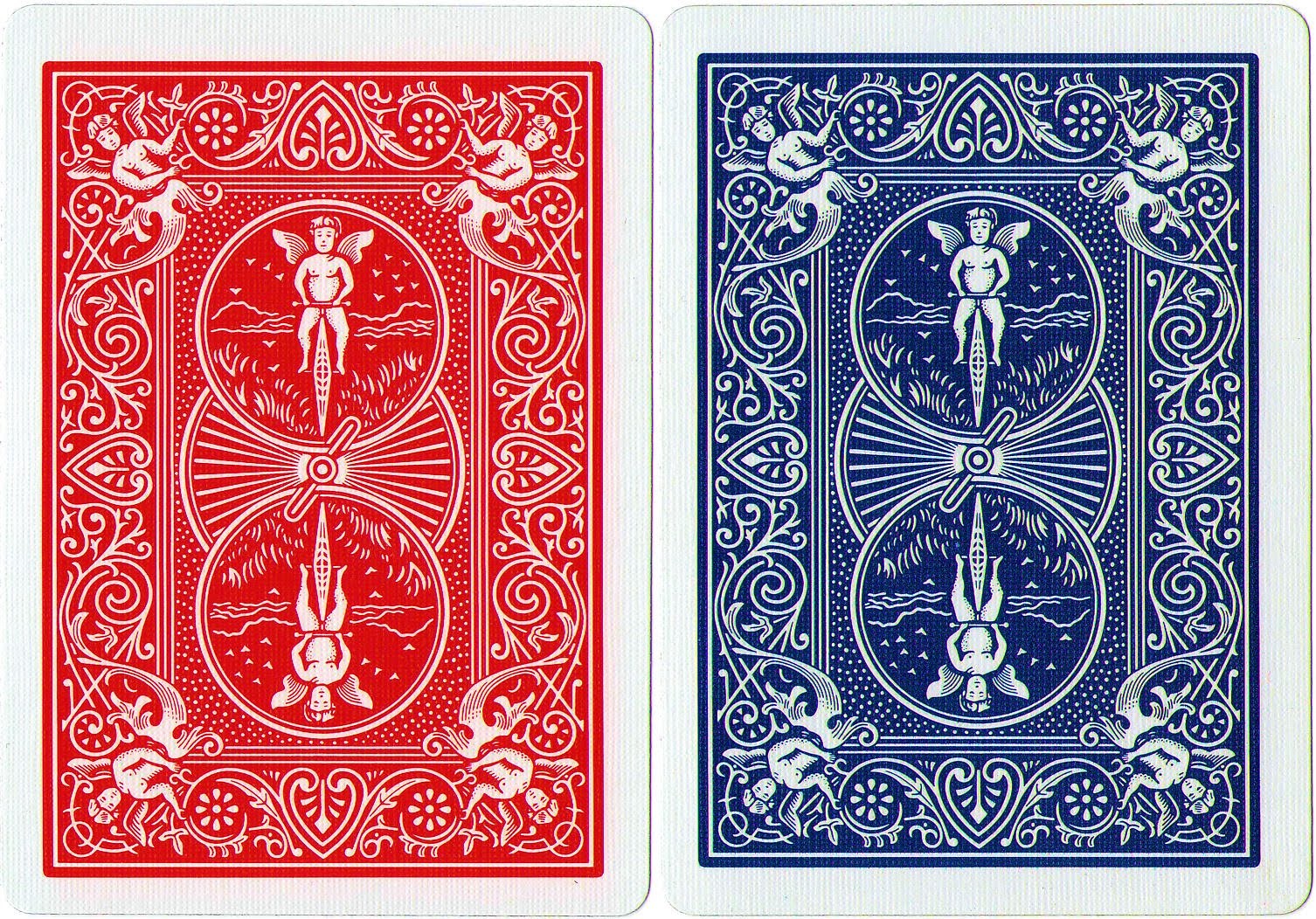This image depicts the back sides of two standard Bicycle playing cards. The card on the left features a red back, while the one on the right showcases a blue back. Both cards display the iconic Bicycle design characterized by a symmetrical, two-way pattern. Central to this design is an illustration of a cherubic, nude angel sitting on a bicycle, surrounded by scenic elements such as grass, mountains, and flying birds. Additionally, each corner of the cards features smaller illustrations of angels, creating a mirrored effect across the entire design.

The cards boast an air cushion finish, giving the surface a textured, lined appearance that minimizes friction, making them ideal for fanning and cardistry. The blue-backed card has a deep sea blue hue, slightly darker than a standard navy, with all details rendered in white lines. Similarly, the red-backed card has a rich, reddish-orange background with white line details. Notably, there is a faint yellow marking on the far right side of the blue card.